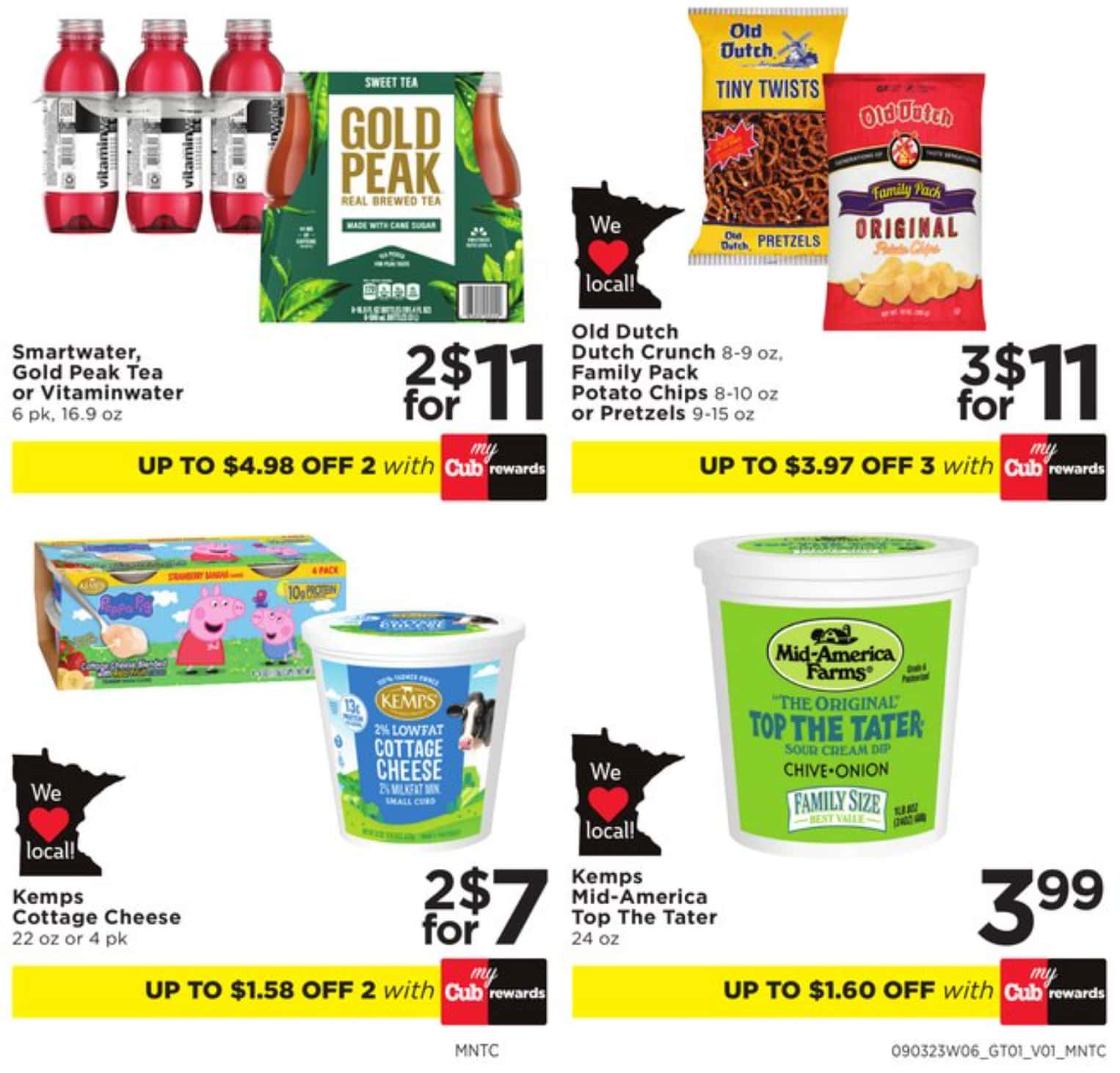At first glance, this appears to be a promotional flyer from a supermarket offering various deals and vouchers. Four items are highlighted for sale:

1. **Smartwater, Gold Peak Tea, or Vitaminwater**: Available in this deal at two for $11, allowing savings of up to $4.98 with the utilization of two My Cub rewards. This offer is prominently displayed with a yellow banner at the bottom. Noteworthy is the red-bottled Smartwater and the Gold Peak Tea which is presented in a green box with gold lettering.

2. **Old Dutch Dutch Crunch Family Pack - Potato Chips or Pretzels**: This deal offers three packs for $11, with a potential saving of $3.97 on the purchase of three using My Cub rewards. The flyer includes the weight details for these items.

3. **Kemp's Cottage Cheese (22oz or Four-Pack)**: Priced at two for $7. Interestingly, one of the packs is themed with Peppa Pig, appealing perhaps to younger customers.

4. **Kemp's Mid America Top Potato, Tried and Onion Flavor**: This single item is priced at $3.99 with no accompanying promotional deal.

The flyer serves as an informative and appealing guide for shoppers looking for value deals on beverages and snacks.